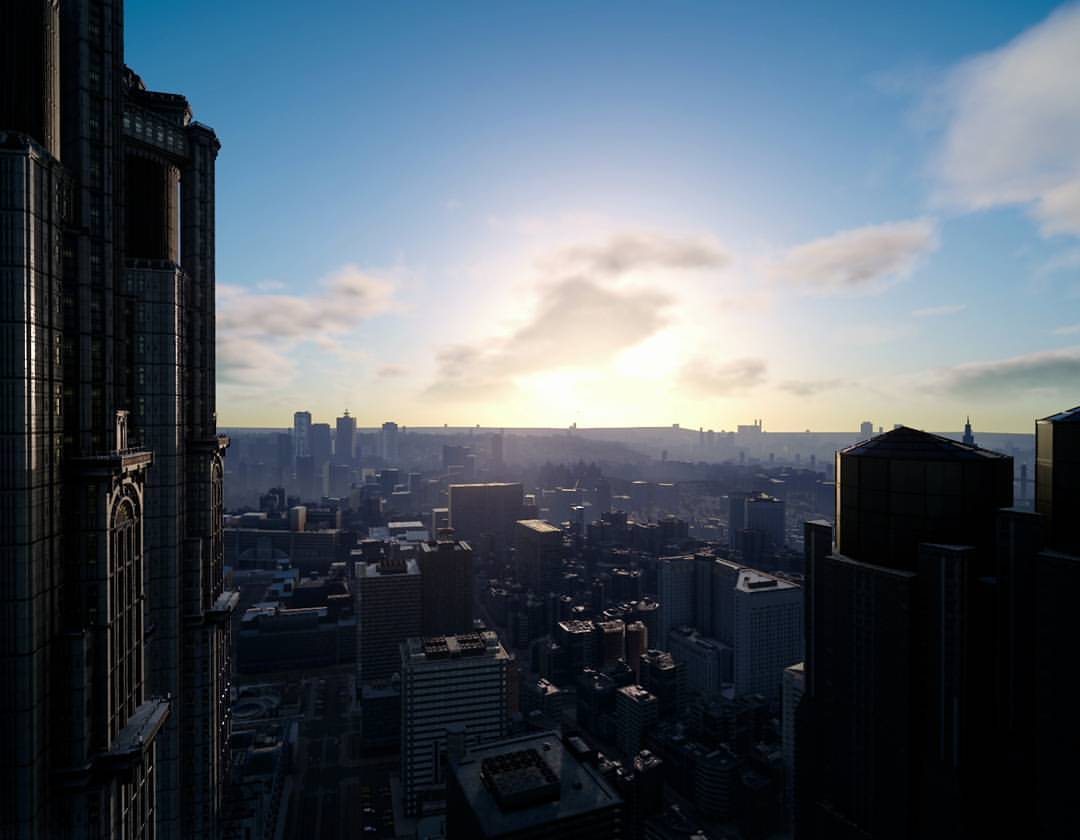Captured from an elevated vantage point, possibly from inside a building or via a drone, this image showcases a sprawling urban landscape. Dominating the left side of the frame is a towering high-rise building, its façade characterized by dark tones and large, arched windows, though it extends beyond the image's boundaries. Stretching into the distance, the cityscape reveals a dense congregation of varied structures, with some buildings showcasing lighter hues amidst the skyline. The horizon glows with the warm, golden tones of either a sunrise or sunset, blending into a brilliant white that highlights a few scattered clouds. Above this, the sky clears to a pristine blue, providing a stunning backdrop to the interplay of light and architecture below.